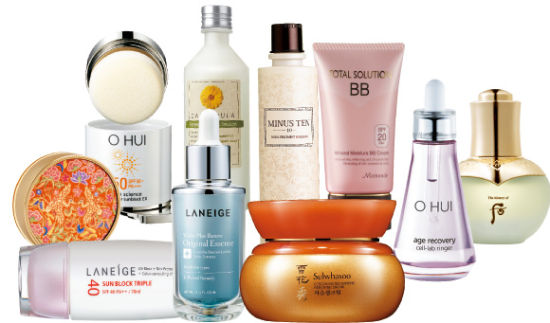This image showcases a diverse array of beauty and skincare products, primarily featuring Korean brands. The collection includes at least a dozen items, spanning facial cleansers, moisturizers, sunscreens, BB creams, and serums. 

From left to right, starting in the bottom left-hand corner:
- A tube of Laneige Sunblock Triple 40 is laying on its side.
- To its right, there is a light blue dropper bottle from Laneige, which appears to be a facial oil.
- Next to this is a large, orange jar of an unspecified product, likely from the brand SWHWAOO.
- Continuing to the right, there is a bottle labeled "O HUI" Age Recovery Serum.
- Near the center, a perfume bottle is visible.
- To the left of the perfume, there's a BB cream.
- In the very middle of the arrangement, there seems to be a cleanser or possibly a bath oil.

The composition of products in this image reflects various aspects of a comprehensive skincare regimen, emphasizing both daily maintenance and specialized treatments.